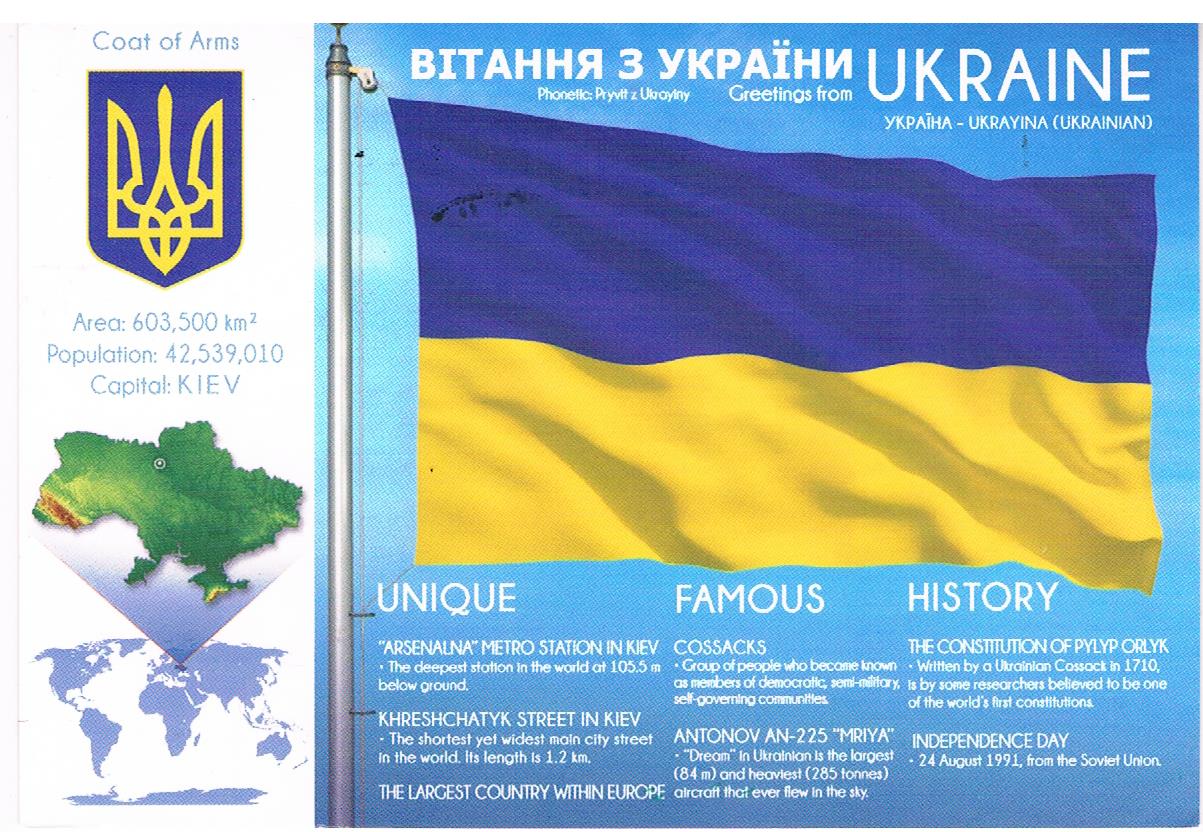The image is a detailed fact sheet about Ukraine, prominently featuring its flag with blue on the top half and yellow on the bottom, fluttering against a bright blue sky. Attached to a silver flagpole, this flag is central to the image. To the right, there is a section providing comprehensive information: the coat of arms in blue and yellow, details of Ukraine's vast area of 603,500 square kilometers, a population of 42,539,010 people, and its capital, Kiev. Alongside, a green map of Ukraine is highlighted on a smaller world map to indicate its location. Notably, the image details Ukraine as the largest country within Europe and mentions the Arsenalna metro station in Kiev, the deepest in the world at 105.5 meters below ground. Historical highlights include Ukraine's Independence Day on August 24th, 1991, from the Soviet Union, and the pioneering Constitution of Philip Orlik in 1710, an early democratic constitution. The words "unique," "famous," and "history" segment the fact sheet, each accompanied by detailed paragraphs expanding on these themes.